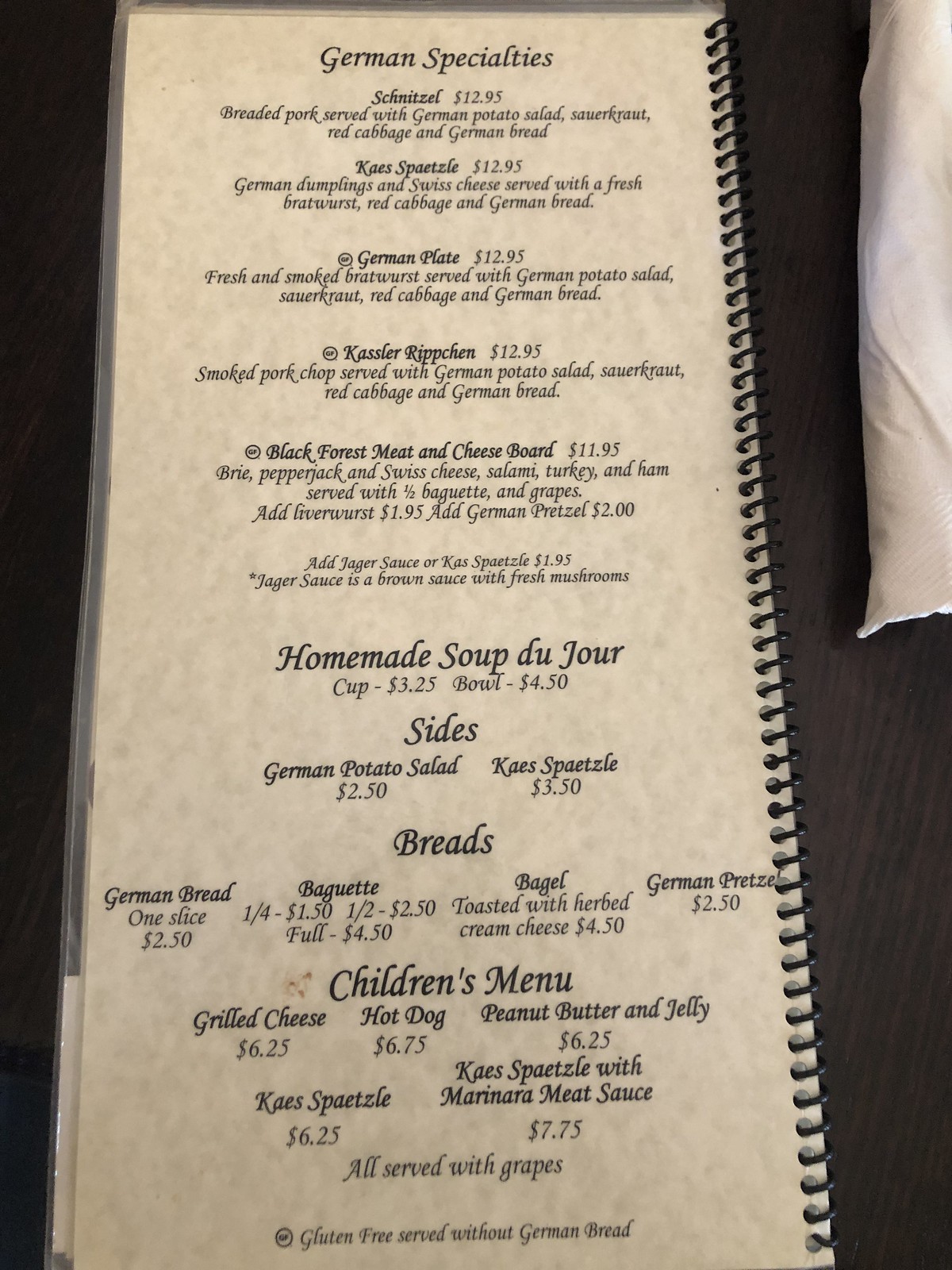The image is a detailed photograph of a restaurant menu, prominently titled "German Specialties" in bold black text at the top. Below this title, the menu lists a variety of dishes, each with specific descriptions and prices displayed in a cursive font. 

At the top of the list is "Schnitzel," followed by a dish described as "German dumplings and Swiss cheese served with a fresh bratwurst, red cabbage, and German bread." Next, under the heading "German Plates," the menu features items such as "Casper Ripschen" and "The Black Forest Meat and Cheese Board."

Further down, another section is titled "Homemade Soup du Jour," indicating the daily soup offering. Following this, the menu lists "Sides," "Breads," and a "Children's Menu."

At the very bottom of the menu, it notes "Gluten-free served without German bread," marked with a small circle to the left, resembling a legend symbol on a map.

Each of these sections, titles, and descriptions are accompanied by prices, all elegantly displayed in a cursive typeface.